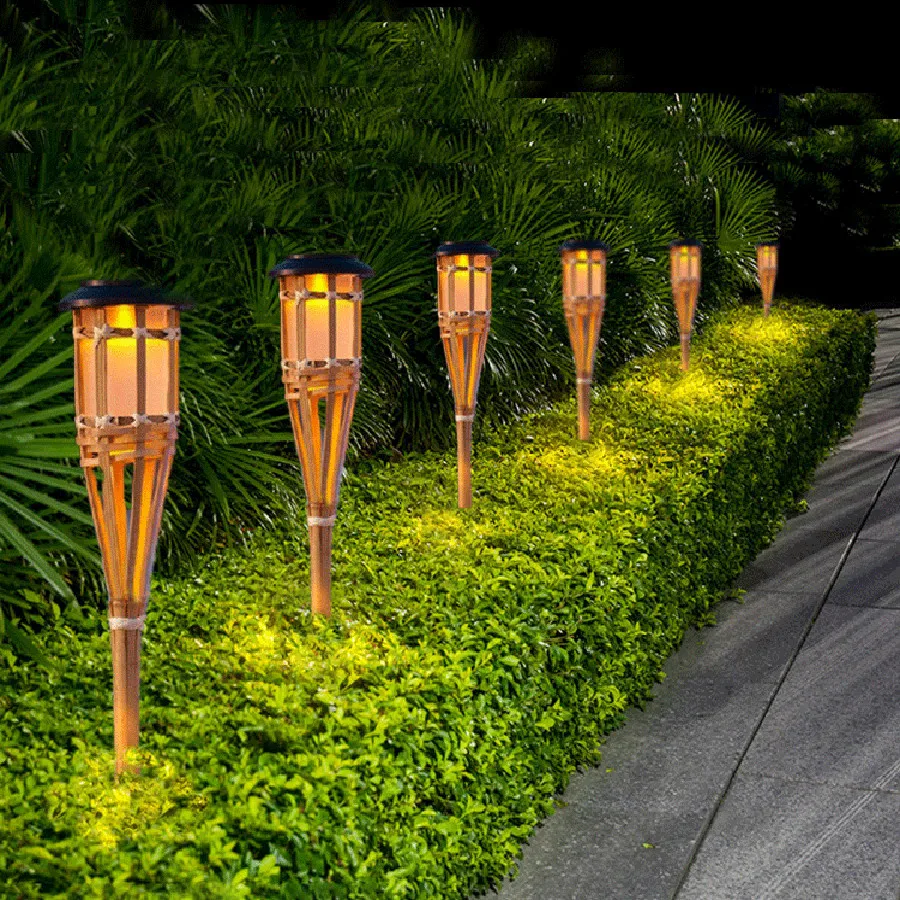The image depicts a nighttime scene featuring a sidewalk made of gray bricks, viewed from a side angle. Running parallel to the sidewalk is a dense hedge showcasing a variety of green shades, including light green, dark green, and yellow-green leaves. Embedded within the hedge are six wooden posts that resemble bamboo lanterns. Each of these posts supports a lit candle at the top, protected by a small black cap. Behind the hedge, thick palm leaves can be observed, and further back, the landscape is filled with tall, straight tree branches, barely visible against the backdrop of a pitch-black night sky.